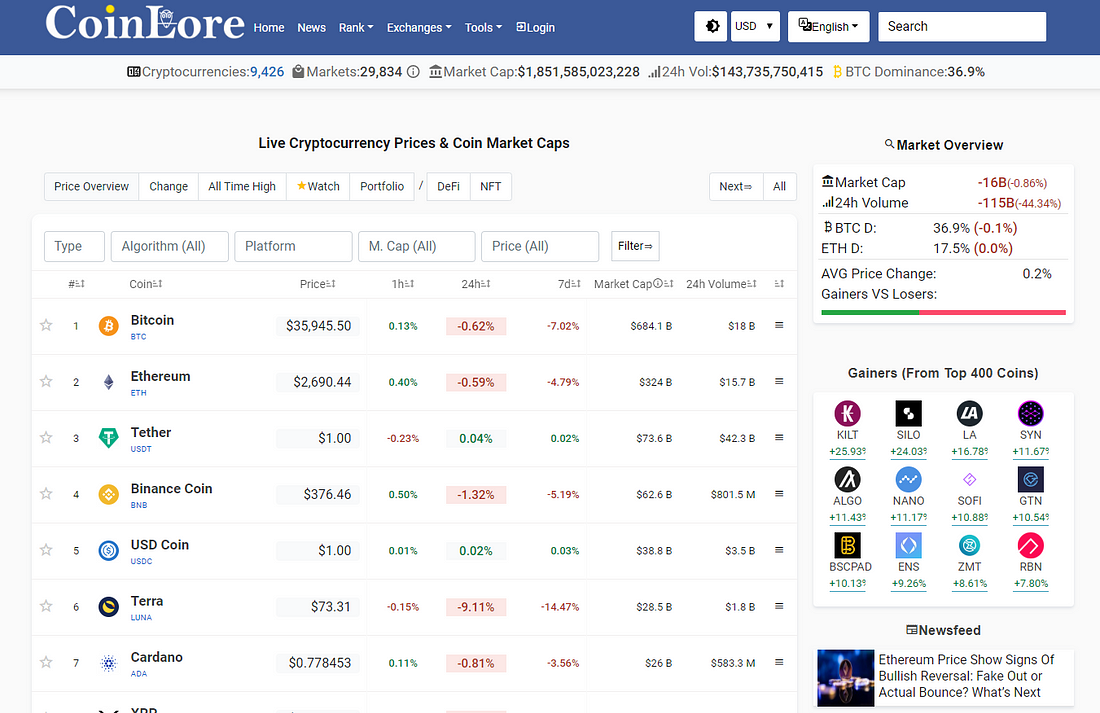**Screenshot from CoinLore Website**

This screenshot, taken on a desktop or laptop computer, captures the CoinLore website, specialized in cryptocurrency information. At the top of the page, a blue banner prominently displays the CoinLore logo in the upper left corner. Next to the logo are navigation buttons, leading to different sections of the site: Home, News, Rank, Exchanges, Tools, and Login. Towards the right side of this banner, users have access to a dark mode and light mode toggle switch, a currency drop-down menu, a language drop-down menu, and a search bar for easy navigation.

Beneath the blue banner, a white banner provides key statistics in black text, listing the following: "Cryptocurrencies 9,426," "Markets 29,834," and "Market Caps 1,851,585,000." To the right of these statistics, additional data points include a "24-hour Service" label and "BTC Dominance: 36.9%."

The main content of the webpage focuses on live cryptocurrency prices and includes several important features: price overview, percentage change, all-time highs, watch portfolio options, and NFT buttons. Below these features is a detailed list of the highest value cryptocurrencies. The list includes major players in the cryptocurrency market such as Bitcoin, Ethereum, Tether, Binance Coin, USD Coin, and Terra, providing a snapshot of their current market standings.

Overall, this screenshot offers a comprehensive look at the CoinLore website's layout and the extensive cryptocurrency data it provides.